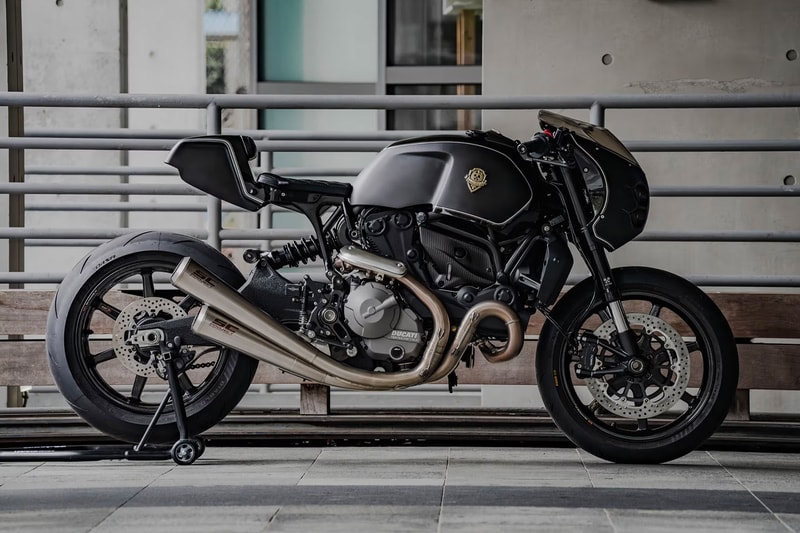This photograph showcases a Harley-Davidson motorcycle elegantly positioned in front of a steel openwork railing, resting on a gray stone pavement. The motorcycle is captured in profile, prominently displaying the distinctive Harley-Davidson gold logo emblazoned on the black metal section just ahead of the steering column. The front is equipped with a sleek black windshield. The intricate brake mechanisms and gears are visible on both the front and rear tires, with the rear tire notably larger. The kickstand is deployed near the rear tire. Noteworthy are the striking golden exhaust pipes, prominently large, running from the motor to the back wheel. In the background, a cement wall and windows provide a glimpse into the interior of a building, adding to the urban landscape.